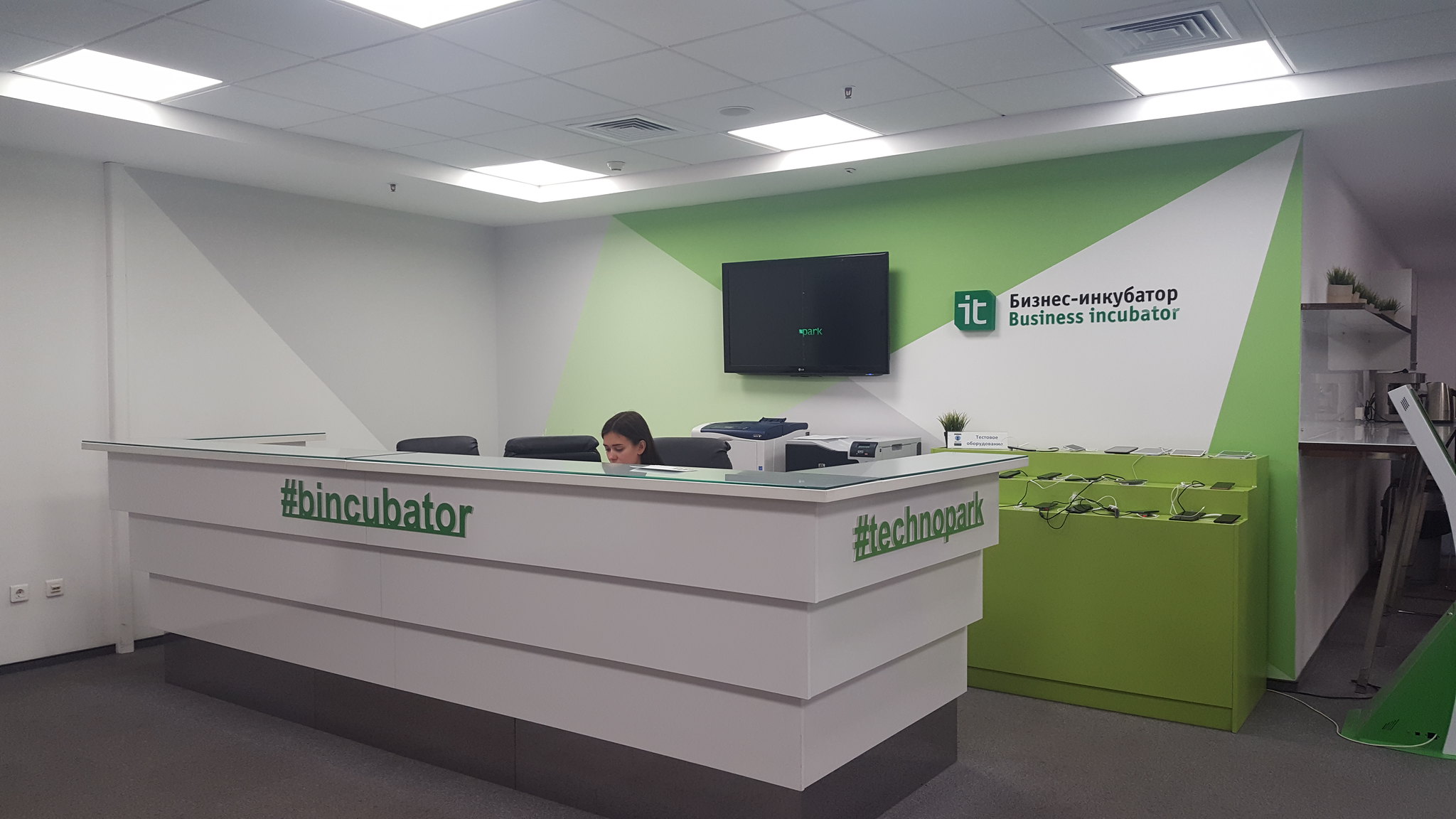This image showcases the reception area of an office lobby, centered around a large white desk. Seated behind the desk is a young woman, who appears to be Asian, with long black hair. The desk prominently displays two hashtag phrases: "#Bincubator" and "#Technopark," which signify the business incubator and technological park aspects of the establishment.

In the background, behind the woman, there is a flat-screen TV mounted on the wall, currently featuring just a black screen. The wall also carries the words "Business Incubator" and some text in what seems to be Russian. There are green-patterned shelves on one side, lined with what look like various mobile devices, adding to the tech-oriented theme of the space. The area is functionally designed with black office chairs and printers, reinforcing the professional, startup-friendly atmosphere of the business incubator.